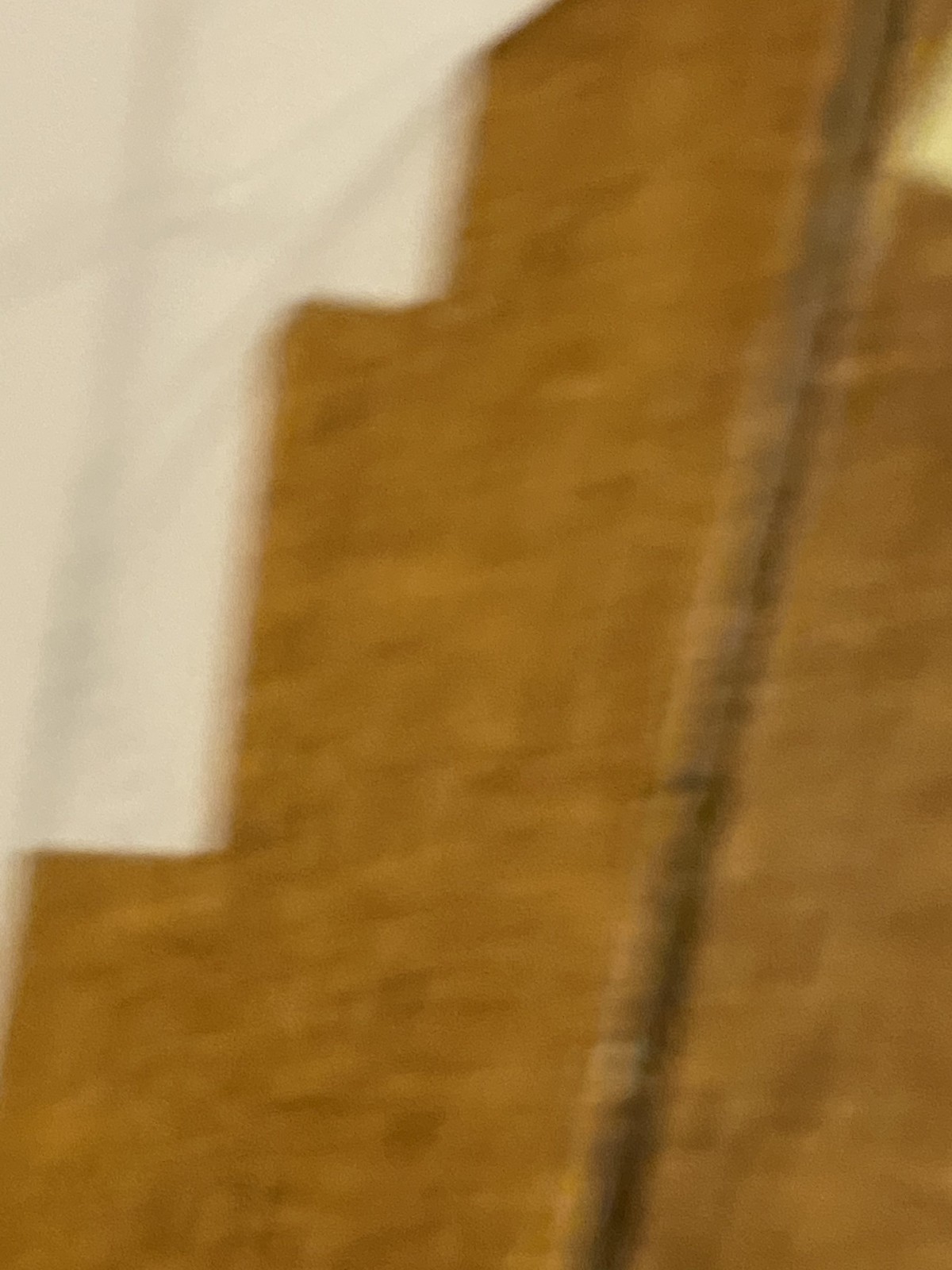A blurry, close-up photograph in portrait orientation predominantly features an orangey-brown wall with a stepped pattern covering around 70% of the image. Positioned towards the right side, a slightly lighter brown pipe runs vertically through the scene, casting a long, gray shadow from the bottom to the top. The brown pipe contrasts with the rest of the wall due to its darker hue. In the upper left corner, there's an off-white area, possibly another wall, with faint vertical, horizontal, and diagonal gray lines. The entire photo appears to be a tightly framed shot of an indeterminate brown material, possibly wood, with tiered formations that resemble steps but are too widely spaced to serve that function. The image's lack of clarity makes it challenging to decipher the exact subjects.